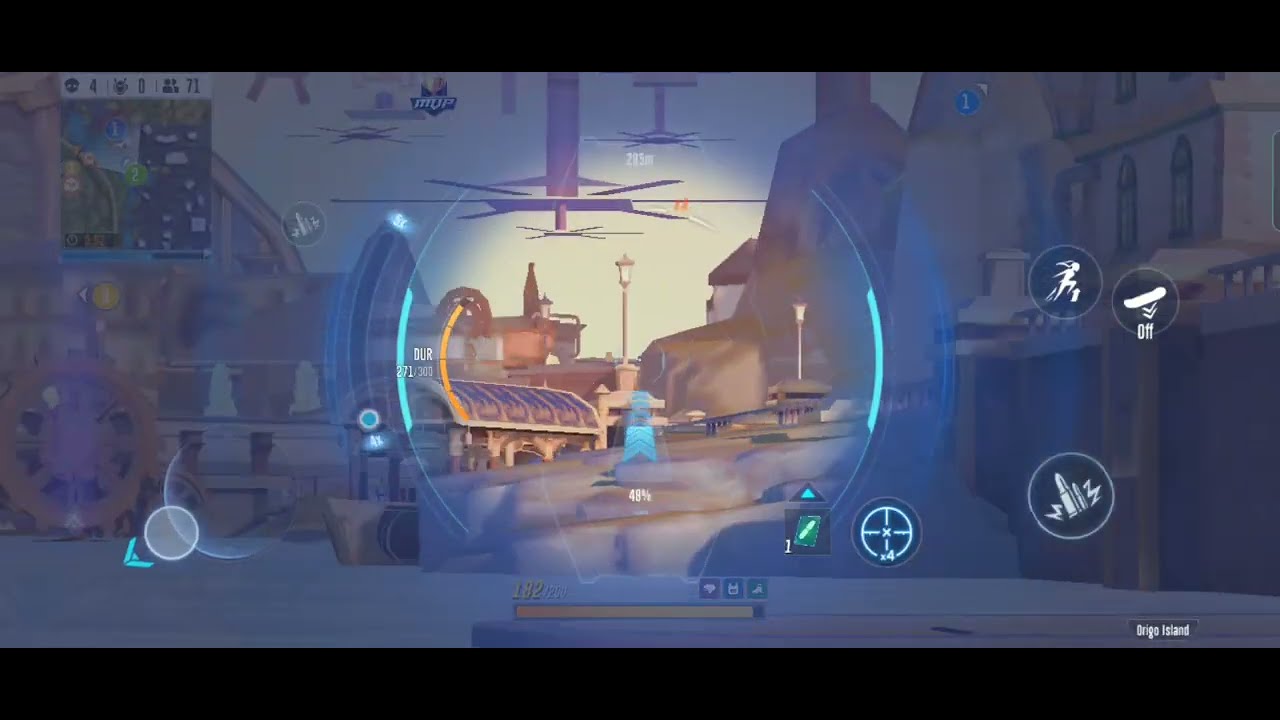The image depicts a game interface on a computer screen, potentially viewed through a VR headset, set within a virtual environment reminiscent of a Star Wars: Return of the Jedi scene, characterized by grays, browns, and brown structures. The interface features a central, well-lit circular area, with the surroundings slightly darkened or blurred for emphasis. Overhead, ceiling fans hang from the top of the image, adding to the immersive atmosphere. Streetlights and various buildings trace out a town or station scene, with some structures appearing to have an oval-shaped, rounded top.

To the right of the circle, there are several icons: one depicting a human-like figure running, another that looks like a hot dog with bees around it, a third showing a bullet, and the closest to the circle, a crosshairs symbol. Additionally, there appears to be some sort of aircraft, possibly an unconventional helicopter, with blades on the bottom and a tube emerging from the middle, indicating 48% in the center. On the left side, in the upper corner, there's a square that could be a map related to the game, while in the bottom left corner, there's another lit-up but blurry circle with a distinct V-shape, akin to the 7 o'clock position on a clock face. This detailed, colorful background injects a lively, highly interactive vibe into the gaming scene.